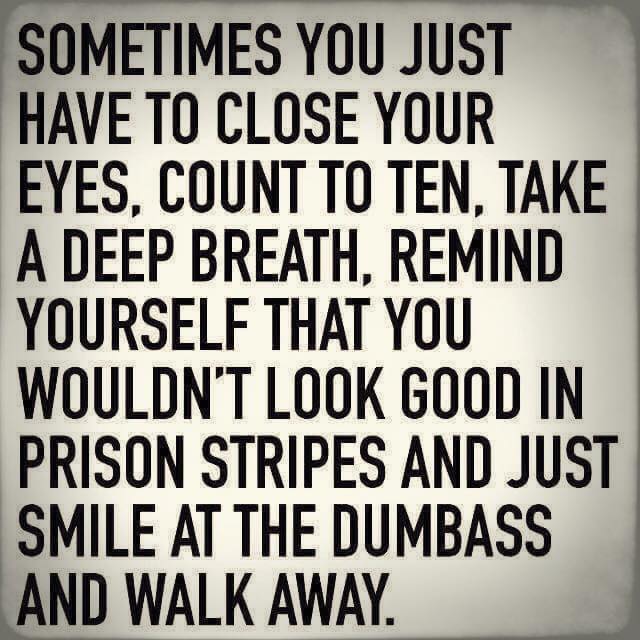The image is a minimalist quote with black, all-caps text on a gray background. The quote reads, "SOMETIMES YOU JUST HAVE TO CLOSE YOUR EYES, COUNT TO TEN, TAKE A DEEP BREATH, REMIND YOURSELF THAT YOU WOULDN'T LOOK GOOD IN PRISON STRIPES, AND JUST SMILE AT THE DUMBASS AND WALK AWAY." The text is evenly spaced, with notable line breaks: "SOMETIMES YOU JUST," "HAVE TO CLOSE YOUR," "EYES, COUNT TO TEN, TAKE," "A DEEP BREATH, REMIND," "YOURSELF THAT YOU," "WOULDN'T LOOK GOOD IN," "PRISON STRIPES, AND JUST," "SMILE AT THE DUMBASS," and "AND WALK AWAY."